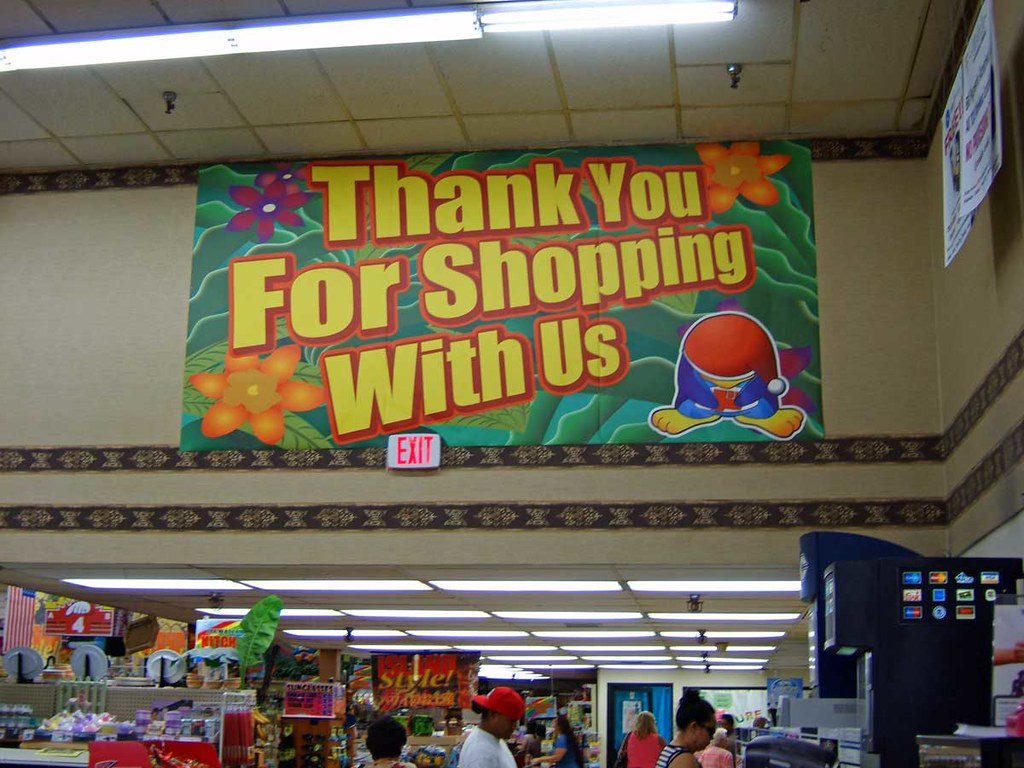The photograph captures the inside of a bustling store, focusing on a large, colorful advertisement on the wall. The banner prominently displays the text “Thank you for shopping with us” in bright yellow letters outlined in red. Surrounding the text are vibrant flowers: orange leaves in the bottom left and top right, and purple flowers with darker outlines in the top left. Green foliage forms a lush backdrop for the banner. In the bottom right corner of the poster, an anthropomorphized blue penguin character with big yellow feet is partially visible, wearing a red Santa hat with a white pompom.

Below the banner, the scene extends to the store interior, where a drop ceiling and shelves filled with a variety of items can be seen. Shoppers mill about, with roughly eight people visible in the middle of the store. To the right, a soda machine dispenses beverages, and an American flag hangs down from the ceiling. The store shelves are stocked with knickknacks, paper plates, decorations including big fake leaves, and more, giving an impression of a party supply store. The photograph's detailed snapshot provides a vivid portrayal of the store's lively atmosphere.